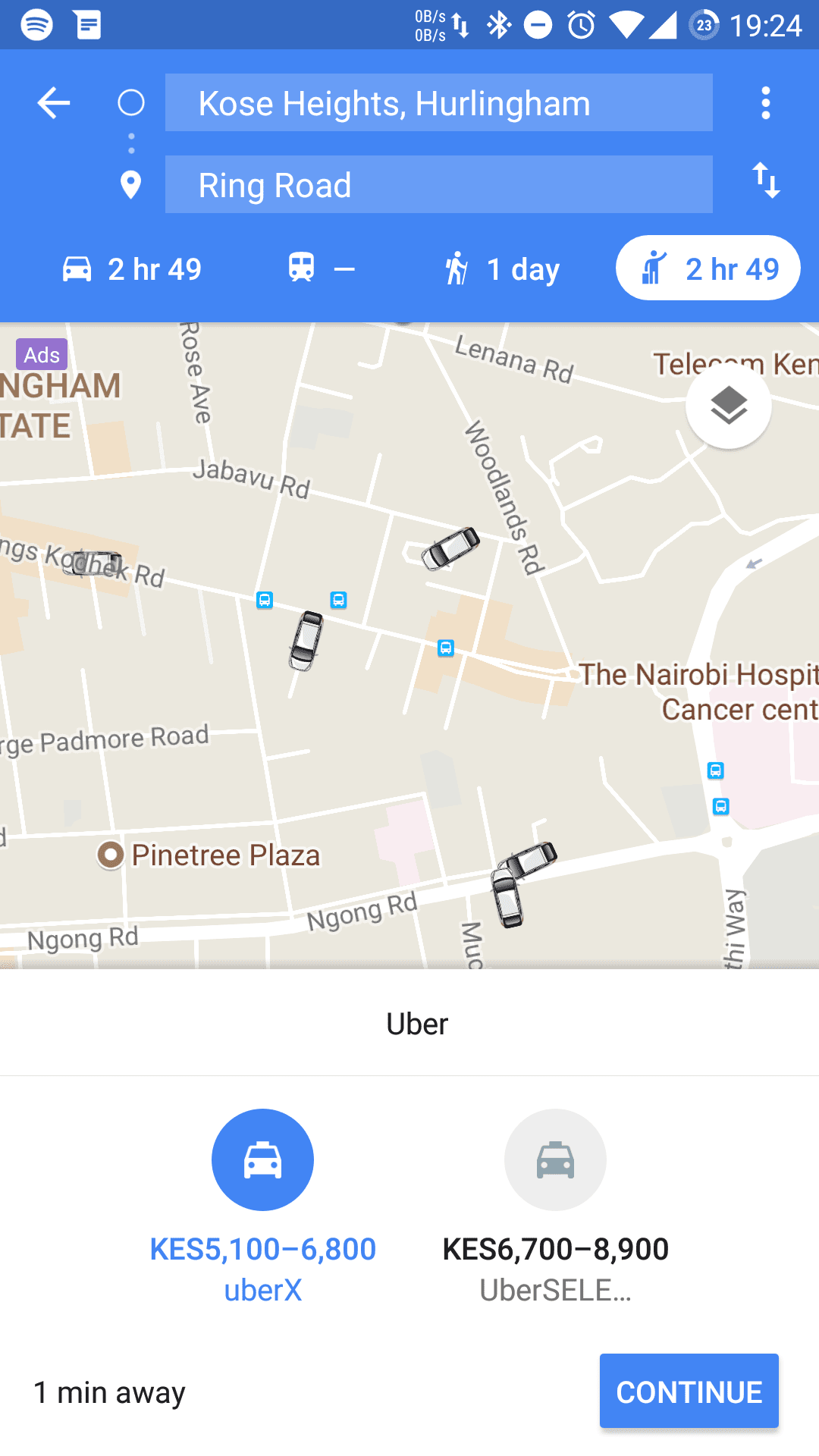In this image, a smartphone is displaying a maps application with intricate details and various features. The top left corner features icons for Spotify and messages, while the top right showcases the time as 19:24, alongside several status indicators: a battery at 23%, network signal, Wi-Fi signal, alarm signal, Do Not Disturb signal, Bluetooth connection indicator, and network speed signal.

The map, colored in grey and white hues with a blue background, highlights "Coors Heights, Halingham" as the current location with "Ring Road" as the destination. The app provides travel times: 2 hours and 49 minutes for driving, the same for hiking, and one day for walking. The map itself displays various roads such as Jabbaw Road, Pine Mall Road, Pine Tree Plaza, Ngong Road, Woodlands Road, and Lenana Road. Landmarks like "The Nairobi Hospital Cancer Center" are also visible, along with several cars scattered across the map.

This maps application, branded by Uber, offers ride options including UberX and Uber Select. The fare ranges from 5100 to 6800 Kenyan Shillings for UberX, and 6700 to 8900 Kenyan Shillings for Uber Select. The app indicates that the nearest vehicle is just one minute away, encouraging users to proceed with a prominent blue "Continue" button located at the bottom right of the screen.